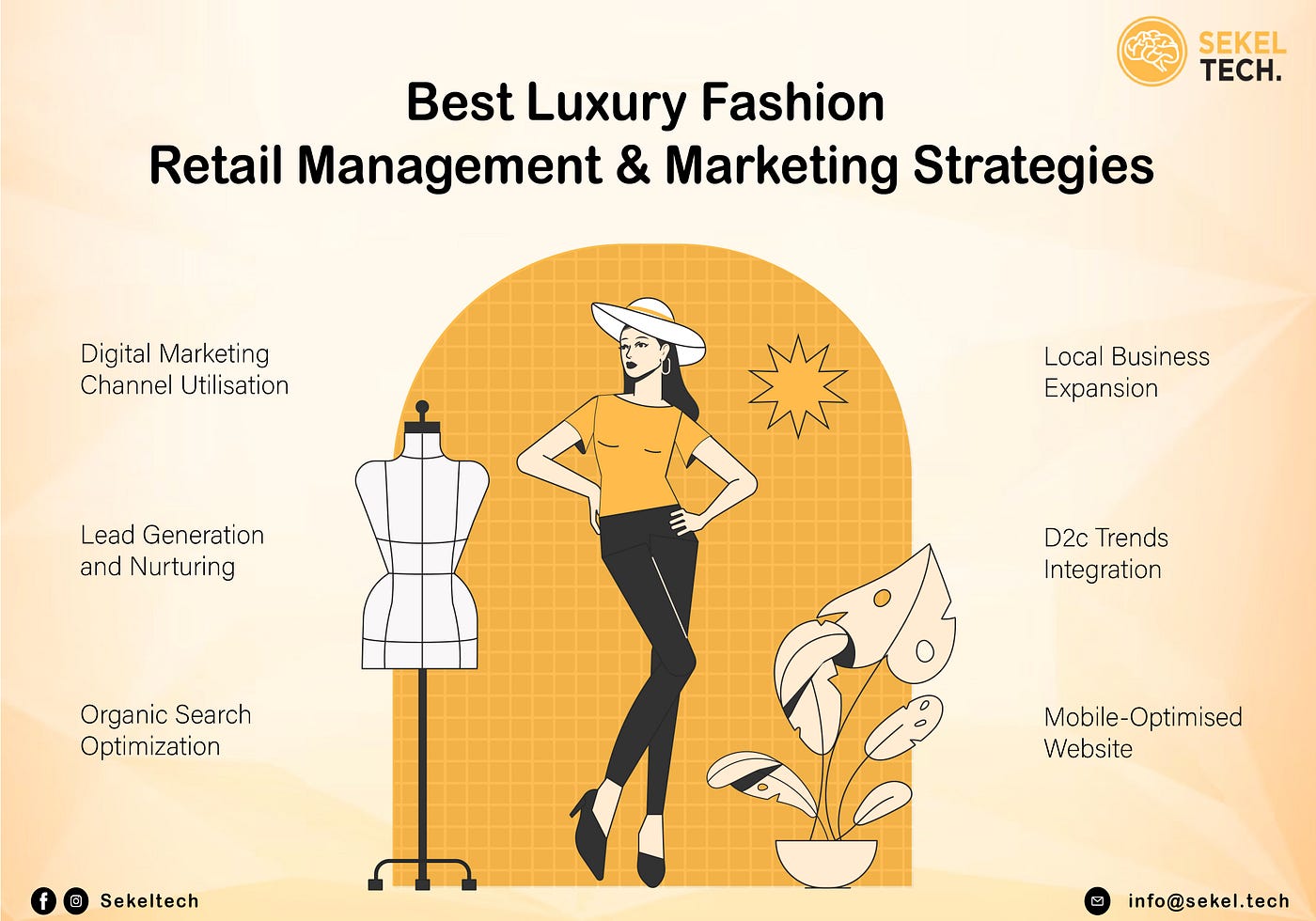A detailed advertising flyer for Sekel Tech with a tan background prominently displays the title "Best Luxury Fashion Retail Management and Marketing Strategies" in large black letters at the top center. The central section features an illustration of a woman posing confidently, wearing a white hat, yellow shirt, black pants, and black shoes. Beside her, there is a mannequin standing on a stand and a potted plant. The left side of the flyer lists key terms such as "Digital Marketing Channel Utilization," "Lead Generation and Nurturing," and "Organic Search Optimization." The right side includes "Local Business Expansion," "D2C Trends Integration," and "Mobile Optimized Website." At the bottom left corner, there are small icons for Facebook and Instagram, along with the name "SEKEL TECH."